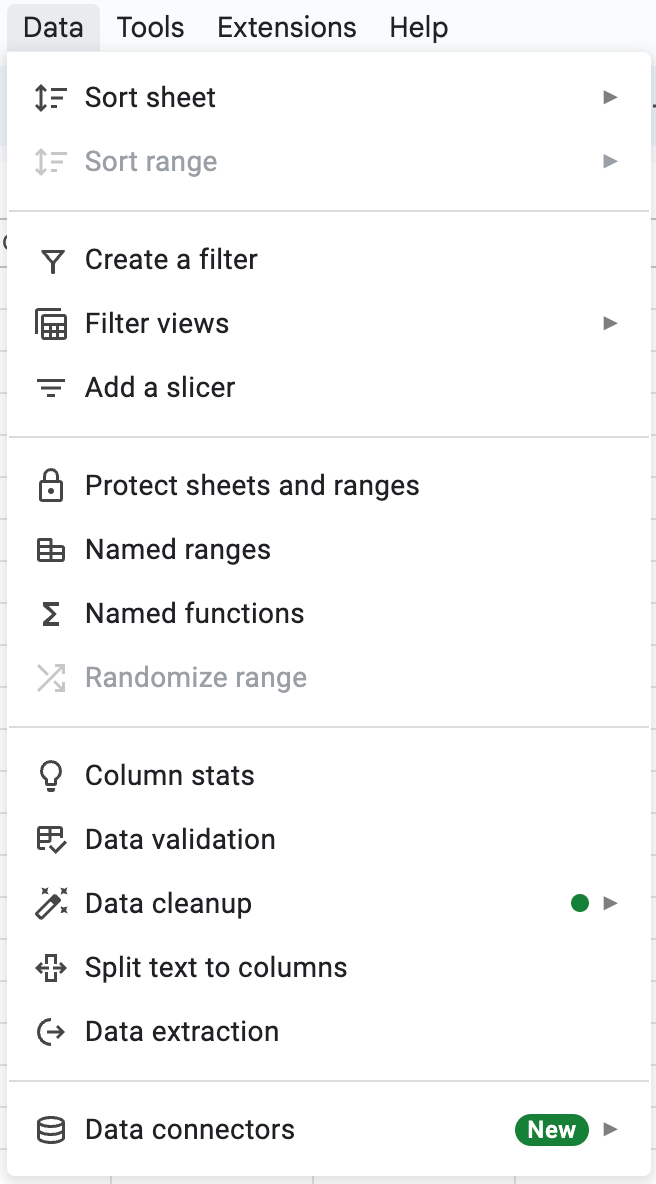A cropped screenshot of a data tab within an app or settings panel, prominently displaying four horizontally listed categories at the top: Data, Tools, Extensions, and Help. The word 'Data' is highlighted in grey, indicating it is currently selected. Beneath it, an extensive drop-down menu is open, extending from the top of the screenshot to the bottom edge, where it is cropped off.

The drop-down menu is organized into several sections:

1. **Sort and Filter Options:**
   - *Sort Sheet*
   - *Sort Range* (greyed out)

2. **Filtering Tools:**
   - *Create a Filter*
   - *Filter Views*, accompanied by an arrow pointing to the left, indicating further sub-options not currently expanded.
   - *Add a Slicer*

3. **Data Management Features:**
   - *Protect Sheets and Ranges*
   - *Named Ranges*
   - *Named Functions*
   - *Randomize Range*

4. **Advanced Data Tools:**
   - *Column Stats*
   - *Data Validation*
   - *Data Clean-up*
   - *Split Text to Columns*
   - *Data Extraction*
   - *Data Connectors*, with a green bubble containing the word 'New' in white text, and an arrow pointing to the left, suggesting additional settings or options available upon expansion.

This detailed breakdown provides a clear view of the structural layout and available functionalities within the data tab of the app's settings panel.